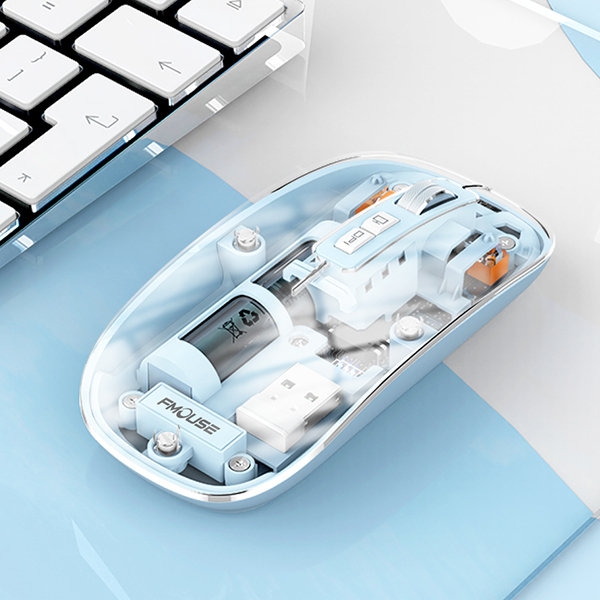The image showcases a highly detailed, possibly computer-generated photograph of the inside of a modern computer mouse. The mouse, which is light blue with a silver border, has its cover removed to reveal an intricate array of internal components. These include a central roller, a battery chamber, several screws, and various inputs, including a place for a USB plug towards the bottom. The branding "F Mouse" is visible on a small blue rectangle inside the mouse.

The background comprises a light blue and white surface. In the upper left corner of the image, part of a computer keyboard is visible. This keyboard features a gray edge, a black base under the keys, and several white keys, including those with upward and right-pointing arrows. The mouse appears to be resting on what seems to be the wrist holder of the keyboard.